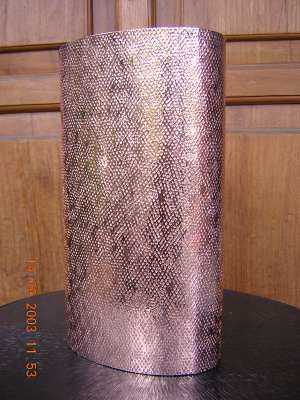In the image, there is a reflective, textured object that has the appearance of a rolled or curved aluminum or possibly diamond-plated steel piece. The material is highly reflective and shimmery, with a texture resembling hammered or molten metal. This object, which could even be mistaken for a fancy, glitzy purse due to its shiny and intricate surface, is placed on its side atop a round, black table. The background reveals wooden cabinetry or a wooden wall, providing a contrasting backdrop to the lustrous item. On the bottom left-hand side of the image, the date "2003" and the figures "1153" or "11 by 3" are displayed in orange text, which appears to be watermarked vertically against the dark table.